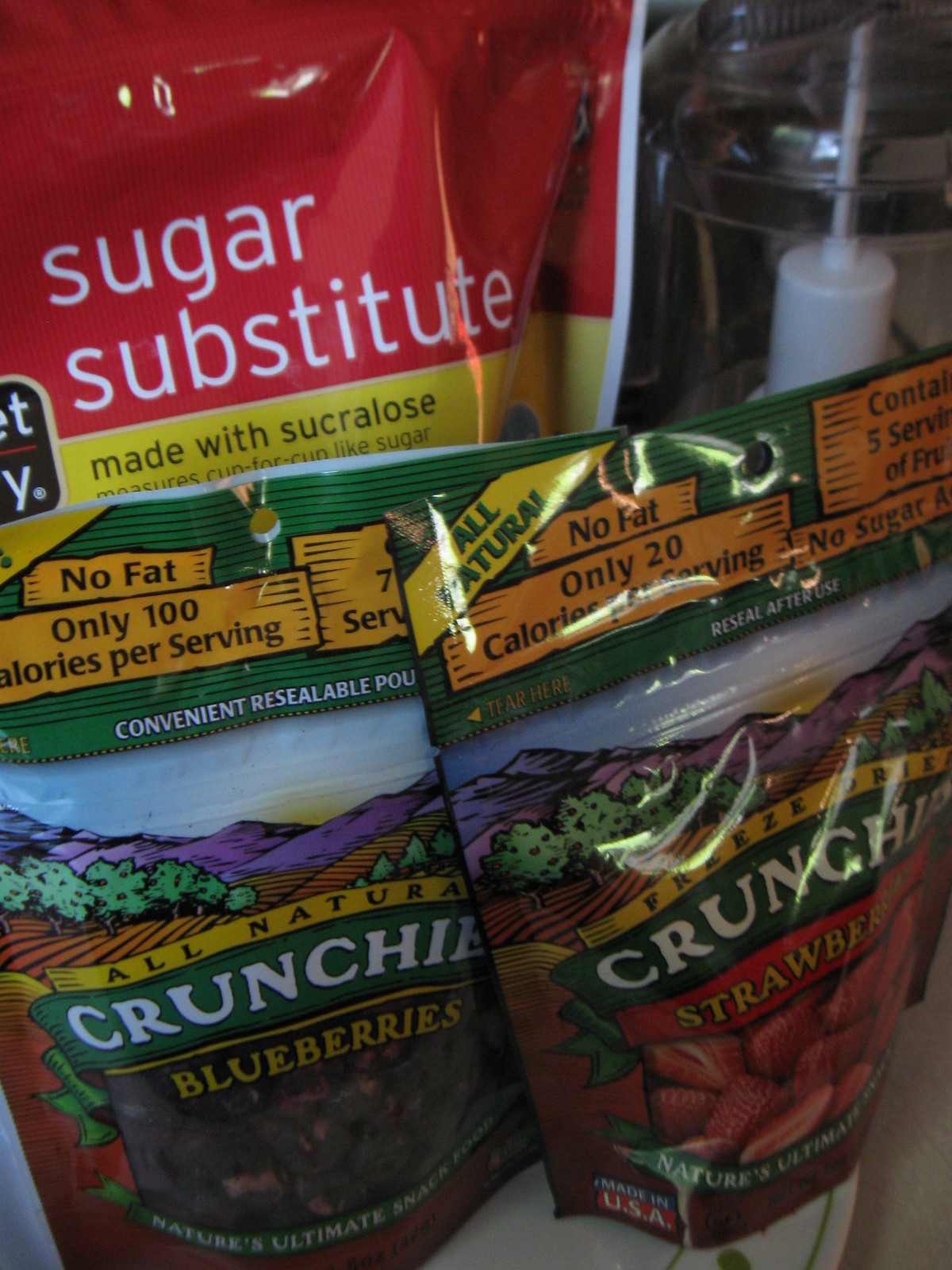This photograph is a detailed close-up of three brightly colored food packages arranged on a round white plate with barely visible green decorations along its borders. In the foreground, two plastic, resealable pouches showcase "all natural crunchy blueberries" and "freeze-dried crunchy strawberries." The blueberry package features a vivid mix of green, black, and orange stripes, with phrases like "no fat," "only 100 calories per serving," and "Nature's Ultimate Snack" visible below a scenic depiction of sky, purple hills, and green fields. The strawberry package mimics this design with similar attributes: "no fat," "only 20 calories per serving," and "contains 5 servings of fruit" highlighted in vibrant orange and red accents. Both packages emphasize their resealable convenience and sport tear marks at their tops.

In the background, partially obscured by the front packages, is a red and yellow sugar substitute package. The top is bold red with white text declaring "sugar substitute," transitioning to yellow where it reads "made with sucralose" and "measures cup for cup like sugar" in black text. The setup is complemented by a suggested kitchen appliance, like a blender or food processor, faintly visible in the background, adding context to the image.